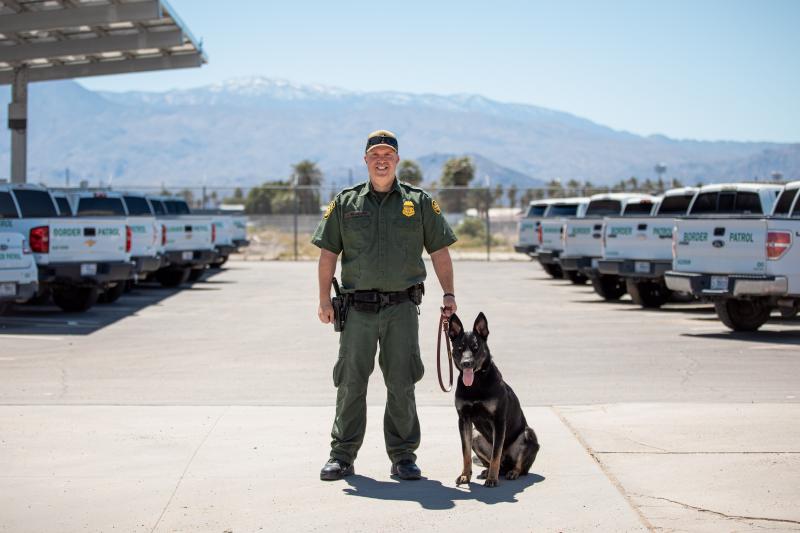The photograph captures a Caucasian Border Patrol agent, identifiable by his full uniform, ball cap, gun belt, and sidearm, standing outdoors in a parking lot. He is smiling at the camera with his black and tan German Shepherd at his right side, the dog’s tongue playfully out. The man, characterized by his beige skin, wears a green collared shirt and dark green pants. The scene is set against a backdrop of a light blue sky, a desert-like mountain range, and some trees. Rows of parked vehicles, including pickups, are seen both to the left and right. The setting depicts the daytime under a clear sky, emphasizing the harmony between the man and his loyal canine companion amidst the rugged outdoor landscape.